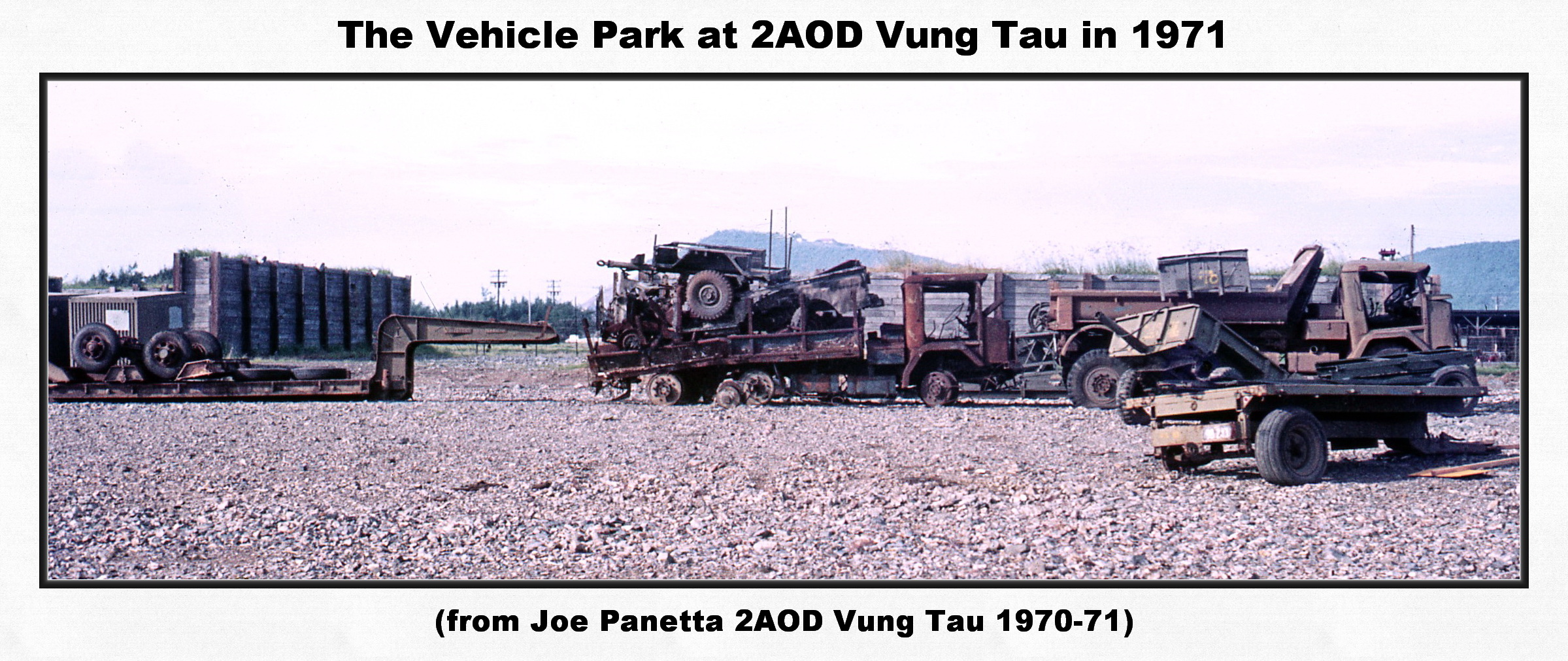This horizontal photograph, titled "Vehicle Park at 2AOD Vung Tau in 1971" in the top text and inscribed "From Joe Panetta, 2AOD Vung Tau 1970 to 1971" at the bottom, captures a collection of worn-down and damaged vehicles, possibly used in the Vietnam War. Sprawled across a gravelly dirt field, these vehicles, including several tanks with prominent large tires, appear aged and inoperable. The backdrop features wooden structures and distant mountains under a very cloudy sky, adding to the somber and historical atmosphere of the scene. The colors in the image range from beige, brown, and gray to black and white, emphasizing the desolate state of the park.